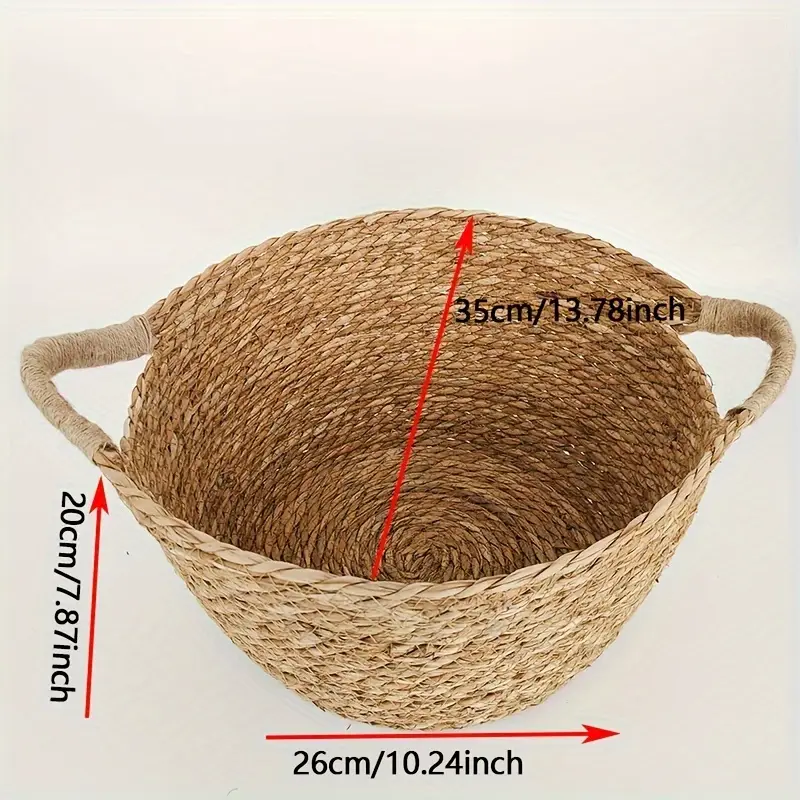The photo depicts a detailed, circular woven basket made of brown jute, with two light brown handles on either side. The basket's meticulous weave pattern is consistent throughout its structure, showcasing a seamless integration of materials. The handles are reinforced with a lighter fabric thread, presumably for better grip. Surrounding the basket are red arrows indicating specific measurements: one inside the basket pointing upwards, marked "35cm / 13.78 inch"; one on the left side pointing to the left handle, marked "20cm / 7.87 inch"; and one at the bottom pointing right, marked "26cm / 10.24 inch". The background of the image is a light gray or beige, highlighting the basket's earthy tones and intricate craftsmanship.